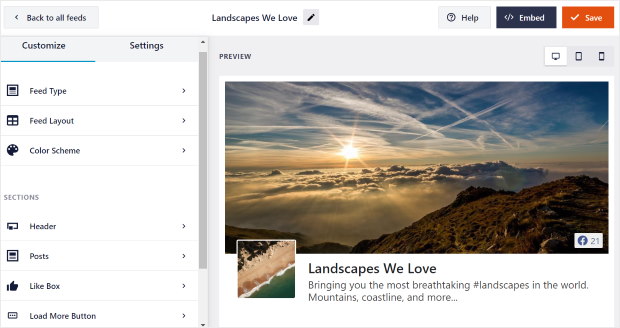This detailed screenshot captures a user interface featuring various customizable settings and editing options for a social media feed. At the top left, there is a "Back to All Feeds" button accompanied by a left-pointing arrow, guiding users back to the main feed selection. The prominent section titled "Landscapes We Love" is highlighted, indicating a focus on breathtaking landscape photography from around the world, including mountains and coastlines.

Several interactive options are visible, such as "Help," "Embed," "Save," "Customize Settings," "Feed Type," "Feed Layout," "Color Scheme," "Header," "Sections," and "Lightbox," providing users with extensive customization capabilities. Each section, including "Header" and "Post," is clearly marked for easy navigation.

Beneath the title "Landscapes We Love," there is an editing pencil icon that suggests the ability to modify this section. A "Load More" button is present, allowing users to view additional content. The interface also displays a "Preview" button for real-time content review, and a Facebook "F" icon followed by the number 21, indicating the post has garnered 21 likes on Facebook.

The highlighted image showcases a stunning photograph taken from the summit of a mountain, offering a breathtaking view above the clouds. The sky is a vibrant blue, with the sun adding a luminous touch to the scene. This "Landscapes We Love" section encapsulates the essence of exploring and sharing awe-inspiring natural vistas from around the globe.